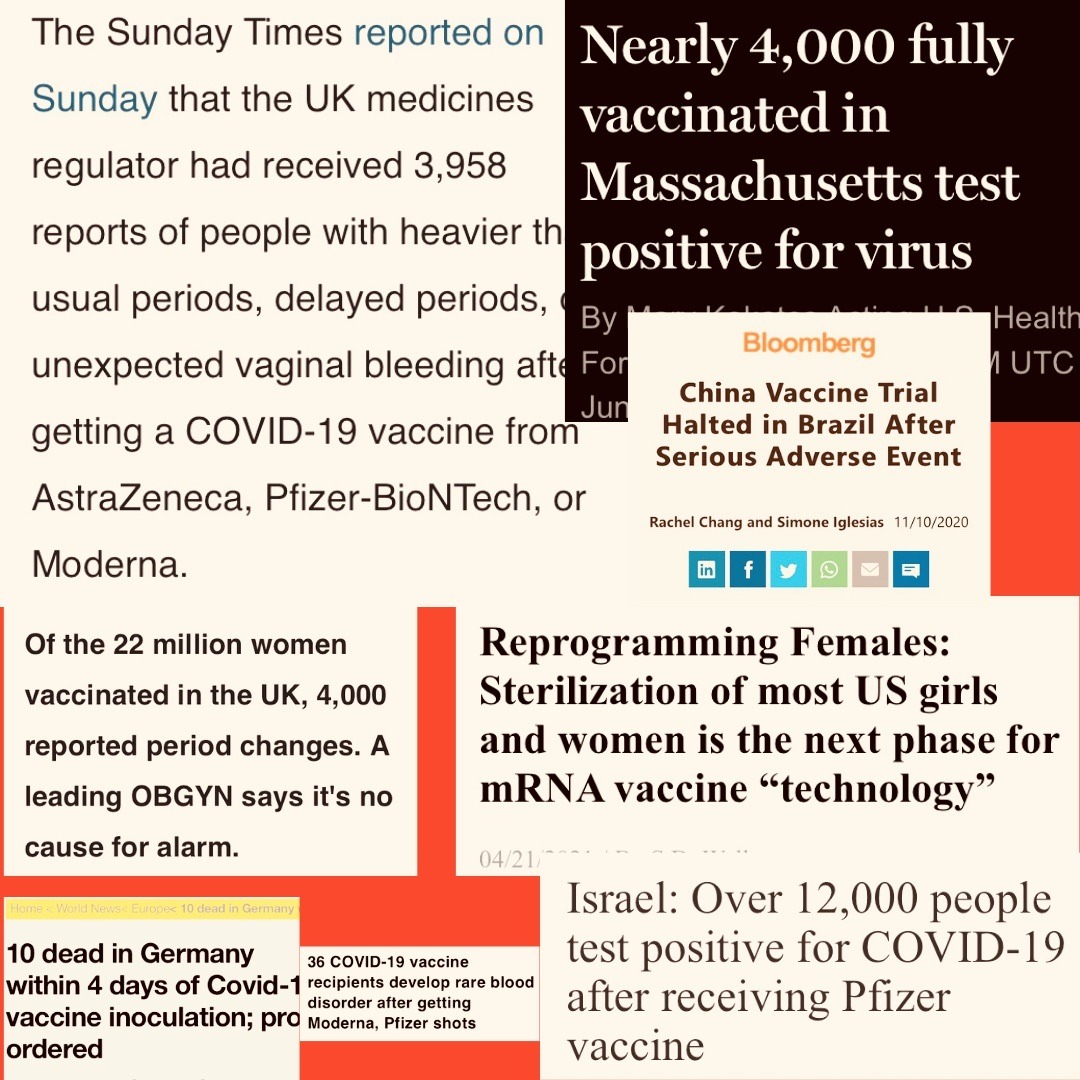The Sunday Times reported that the UK Medicines Regulator received 3,958 reports of women experiencing heavier than usual periods, delirium, and unexpected bleeding after receiving the COVID-19 vaccines from AstraZeneca, Pfizer-BioNTech, or Moderna. Out of the 22 million women vaccinated, approximately 4,000 reported changes in their menstrual cycles. According to a leading OBGYN, these occurrences are not cause for alarm.

In Germany, within four days of COVID-19 inoculation, a father and son reported adverse reactions. Additionally, 36 recipients of the Moderna and Pfizer vaccines developed a rare blood disorder. In Massachusetts, nearly 4,000 fully vaccinated individuals tested positive for the virus.

In a separate incident reported by Bloomberg, a trial of a Chinese COVID-19 vaccine in Brazil was halted due to a serious adverse event. Concerns were also raised about the mRNA vaccine technology and its potential implications for female sterilization in the U.S.

Furthermore, over 12,000 people in Israel tested positive for COVID-19 after receiving the Pfizer vaccine. 

These reports capture a range of reactions and concerns linked to the global COVID-19 vaccination effort.